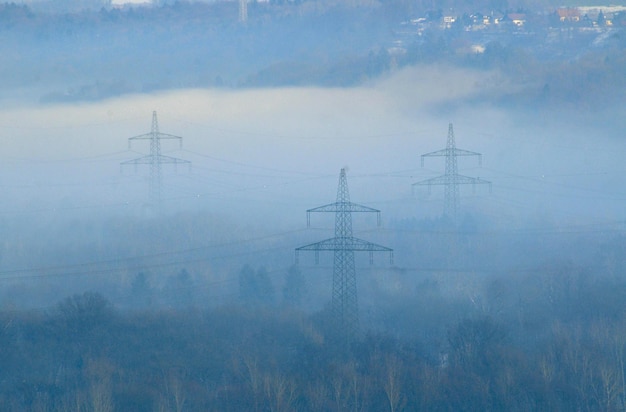This rectangular, landscape-oriented photograph captures a foggy scene taken from an elevated viewpoint. The ground is densely covered in trees and shrouded in thick, light blue fog, which obscures clear visibility and becomes denser as it recedes into the distance. Rising from the fog are three large electrical power towers with wires stretching between them, adding an industrial element to the natural setting. At the top right corner of the image, a small town with houses is visible, seemingly perched on a hill above the blanket of fog. The overall color theme of the photograph is a serene blue, contributing to the misty, ethereal atmosphere of the scene.